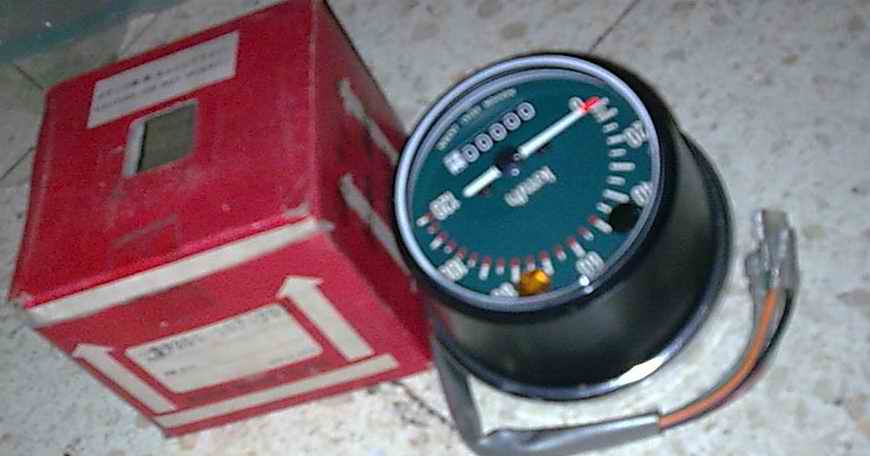A blurry photograph taken with flash, evident from the bright reflection on part of the image, shows an object on a tiled surface that could either be a kitchen counter or a floor. The tiles have a stone effect, featuring a gray base with mottled spots of various colors, resembling a rock filled with different crystals. Dominating the scene is a red box marked with white arrows indicating "this way up" on two sides. The box also has white rectangular labels with illegible information.

Emerging from the box is a round dial, likely a speedometer or a similar counter. The dial's housing is black with a silver ring encircling the analog display. The background of the dial is teal green, and the indicator hand is white with a bright red tip, marked with incremental stages and possibly labeled with "kilometers per hour" in the center. The dial is upside down in the photograph, and at its bottom, a total counter shows zeros. Visible wiring is connected to the device, which rests on the detailed, stone-like tiled surface.